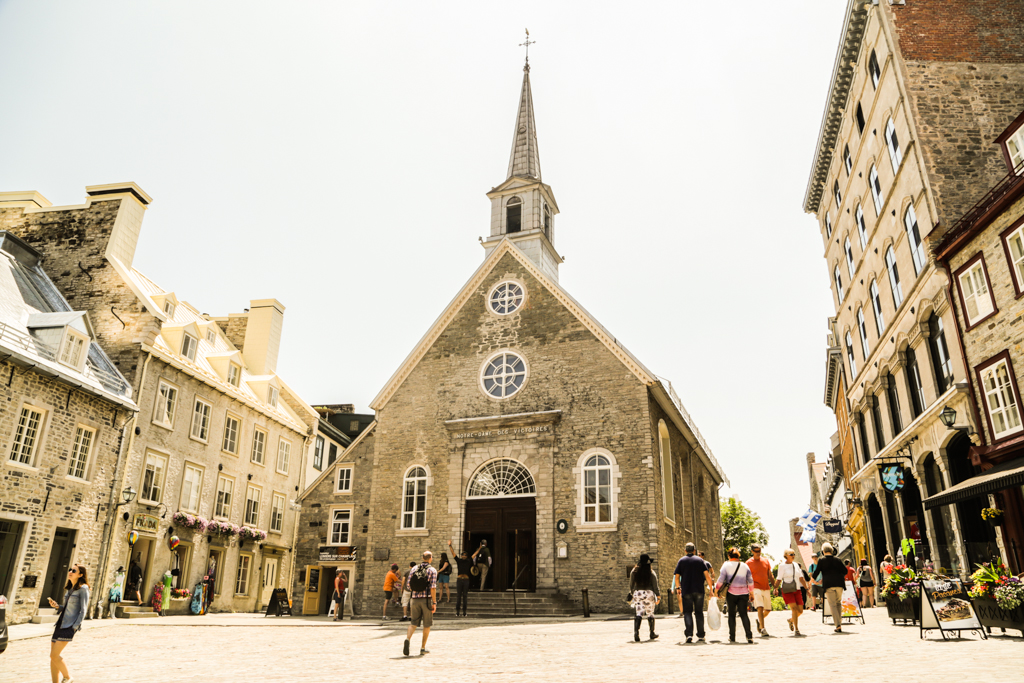The photo captures a picturesque scene of a small tourist town, possibly in Europe. Dominating the center of the image is a grand stone church adorned with a pointed spire and a cross at the top, flanked by two circular windows near its roof. The church is beautifully constructed with gray-brown stone, echoing the old-world charm that permeates the entire setting. Surrounding the church are buildings of the same stone material, with the structures on the left being shorter but wider compared to the taller ones on the right.

A cobblestone or brick street runs through the town, packed with people of all ages, some in shorts indicative of summer. Many are strolling with packages, likely from shopping excursions, while others are either entering the church or simply admiring it. The street is lined with quaint buildings that likely house cafes, pubs, and shops, some adorned with flowers and flags. A couple of trees can be seen in the background, enhancing the picturesque ambiance. The sky above is a pale gray, adding to the serene and timeless atmosphere of the scene.